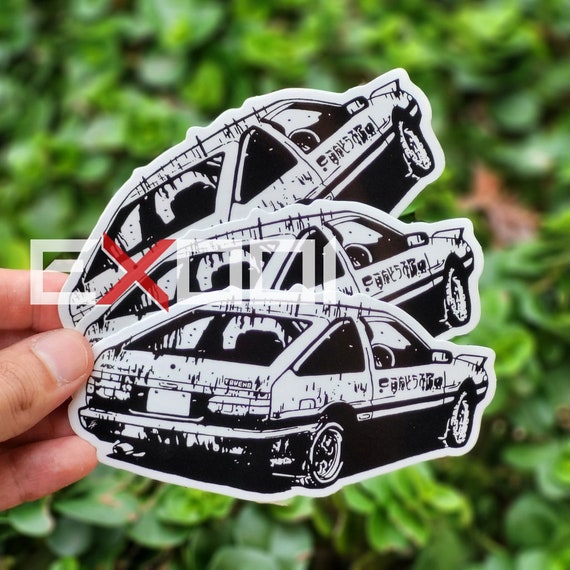A color photograph features a Caucasian hand, visible only by the fingertips on the left side, holding three large black and white stickers, each depicting the rear of an older sports coupe model with a partly busted appearance. These stickers, placed one above the other, show cars with black speckles or mud-like markings. The background is a blurred mass of green leaves, indicating a plant-filled setting. A watermark stretches across the center of the image, with the text "EXOZI" in white letters and a distinctive red 'X'. Additionally, the word 'TROEND' is visible on the back of one car sticker.